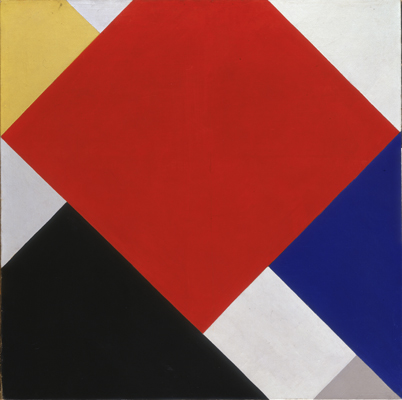This image is a modern abstract composition with a central red diamond, missing its top corner, positioned diagonally. The red diamond extends down about three-quarters of the way and makes contact in the bottom left with the corner of a black square, which is partially cut off. Adjacent to this, towards the right, a white square connects to the bottom edges of the black and red squares, though its lower part is also truncated. Directly below the white square is a small gray triangle, and above it, a blue triangle that intersects with the red diamond as well. In the upper right corner of the image, there is a larger white triangle. In the upper left corner, a yellow square touches the red diamond, with a smaller white triangle next to it. Additionally, midway down the left side of the image, there is another white triangle. The overall effect is a series of angular shapes and intersecting planes, creating a dynamic visual centered around the red diamond. The geometric composition blends the principles of cubism with modernist abstraction, emphasizing fragmented forms and intersections.